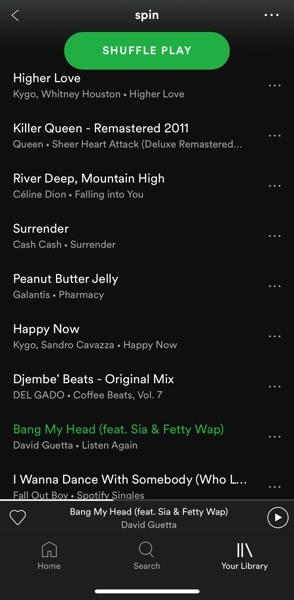The image is a screenshot taken from a mobile device in portrait mode. At the top center, the word "spin" appears in lowercase. Below this, there is a prominent green button with rounded corners labeled "Shuffle Play."

Beneath the Shuffle Play button, there are rows of music selections organized in a single column. The first song listed is "Higher Love," followed by "Killer Queen - Remastered," "River Deep - Mountain High," "Surrender," "Peanut Butter Jelly," "Happy Now," "Djembe Beats," and finally, "I Wanna Dance with Somebody (Who Loves Me)."

In the eighth row, a song called "Bang My Head (feat. Sia & Fetty Wap)" by David Guetta is highlighted in green, indicating the current selection. Directly beneath this highlighted row, it shows partial playback progress for the song "Bang My Head." To the left of this playback information, there is a heart icon which, when selected, marks the song as a favorite. To the right, there is a play button which likely allows the user to either resume or skip forward in the track.

At the bottom of the screen, there are three icons: Home, Search, and Your Library. The "Your Library" icon is highlighted, indicating that this is the current section being viewed.